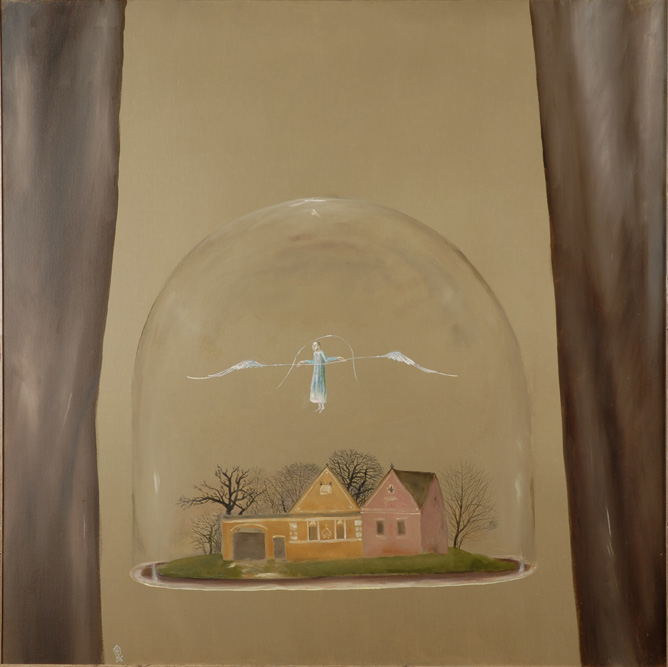This detailed painting portrays a scene within a snow globe-like glass dome against a tan background, bordered by rich brown curtains on either side. The dome, meticulously crafted to imitate glass, features a grassy green area at its base. Inside, two distinct houses are depicted: one predominantly yellow with a brown garage and white-outlined windows, and an adjoining section in soft pink with a peaked roof. Behind the houses stand four barren trees, their branches stark and leafless. Hovering above this quaint setting is an ethereal angel with extended, feather-like wings and a flowing blue gown, adding a touch of celestial beauty to the tranquil domestic scene within the glass enclosure.